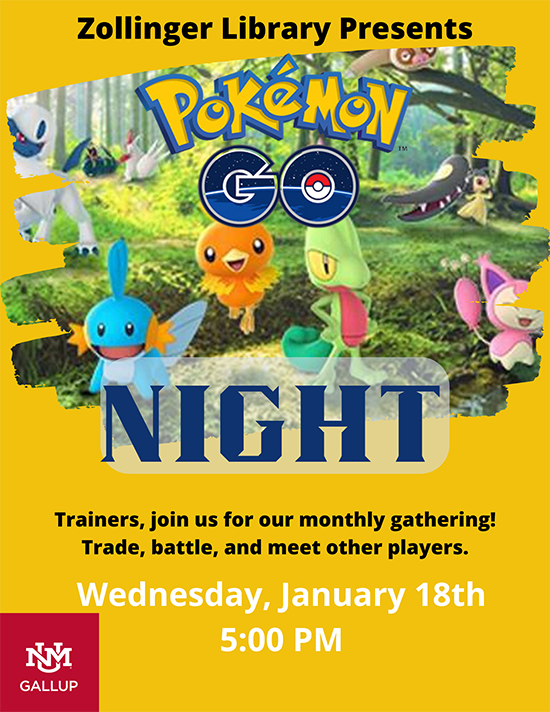Join us for an exciting evening at the Zollinger Library's "Pokemon Go Night"! The vibrant poster, set against a backdrop of mustard yellow, invites Pokemon enthusiasts to a night of fun and adventure. The cheerful design prominently features an array of adorable Pokemon creatures in various colors. Among them, you'll spot a lizard-like Pokemon, a small pink bunny or kitty-like character, an alligator resembling a sloth, and even a robot-like figure in the background. There's also a chicken-like Pokemon with a red crest, possibly a rooster.

Trainers are encouraged to come together for this monthly gathering to trade, battle, and connect with other players. Mark your calendars for Wednesday, January 18th at 5 p.m., taking place at the NM Gallop. The event's details are highlighted in a distinct maroon-colored section on the left-hand corner of the page. Don't miss out on this cute and lively event!